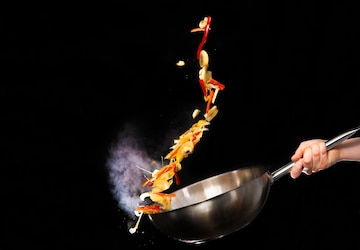In the image, set against a completely black background, a white hand grips the handle of a silver wok pan. The pan is caught in mid-toss, sending a colorful array of vegetables—primarily red peppers, yellow vegetables, white onions, and possibly mushrooms—soaring into the air in a graceful arc. Wisps of white smoke or steam waft off from the lower left side of the pan, enhancing the sense of sizzling heat. The hand holding the pan is the only visible part of the person, emphasizing the dynamic motion of tossing. The sleek, elegant silver wok pan appears to be of high quality, adding to the overall impression of a professional or skilled chef in action.